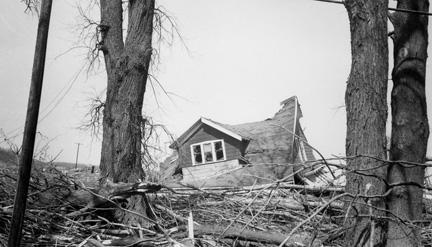A black and white photograph captures a desolate scene dominated by a small, dilapidated house that appears to be collapsing. The house, which is noticeably tilted about 10 degrees counterclockwise, showcases significant decay with its upper windows slanted towards the ground and its right side seemingly torn and ripped. This structural distress gives the impression that the building has been sinking unevenly into the earth, with the right side still somewhat upright while the left side has given way. Surrounding the house is a landscape marked by devastation: the foreground is littered with fallen, dead trees and a chaotic assortment of branches and twigs. At least three tree trunks remain standing; two are situated in the lower right corner, extending upward, and another is slightly left of center. Adding to the eerie atmosphere, one tree notably bifurcates at its top. The overall lack of nearby structures suggests this scene is set in an isolated, possibly rural area, contributing to its forlorn and spooky feel.